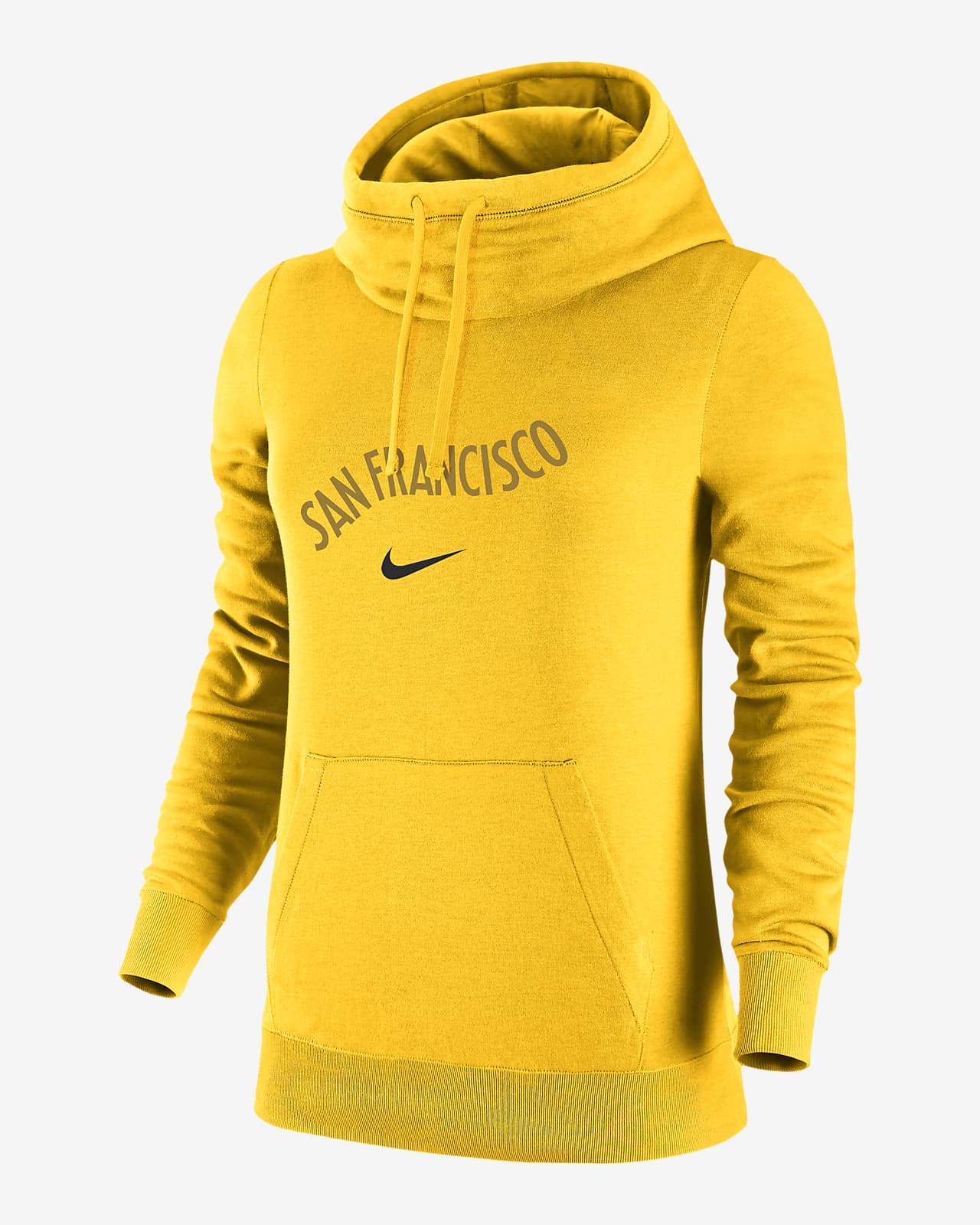This is a professional, color photograph of an athletic, tight-fitting Nike hoodie in a portrait format against a completely white background, making it appear as if it's hovering. The hoodie is a mustard yellow color and features a sleek, thin material with ribbed knit cuffs at the sleeves and bottom. The front of the hoodie sports a wavy, all-caps "San Francisco" text above the iconic black Nike swoosh symbol, set in a black and brownish font. It has a front belly pocket designed for hand placement, visible wrinkling in the fabric around the slightly bent elbows, and a high neck area equipped with two drawstrings for adjusting the hood. The hoodie appears puffed up as if worn, though no model or mannequin is present.